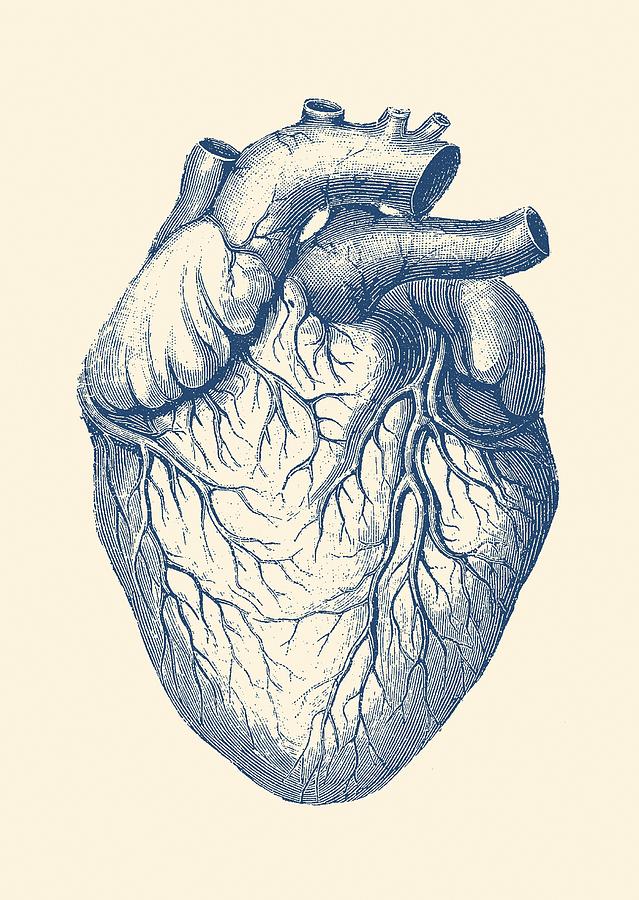This picture is a detailed, computer-generated depiction of a human heart, possibly also representing another animal heart. The heart is rendered with a blue tint against a pinkish-tan background, highlighting its intricate structure. The veins and arteries branch out like tree roots, descending towards the bottom of the image and giving a visually striking effect. The major arteries and veins, characterized by large, open circles, are prominently displayed at the top. These open circles face the right side of the image, suggesting an anatomical orientation. The heart features other smaller vessels branching out, adding to the level of detail. The image showcases the muscular texture of the heart, with numerous lines and intricate details throughout, resembling both a meticulous drawing and a computer-generated graphic.